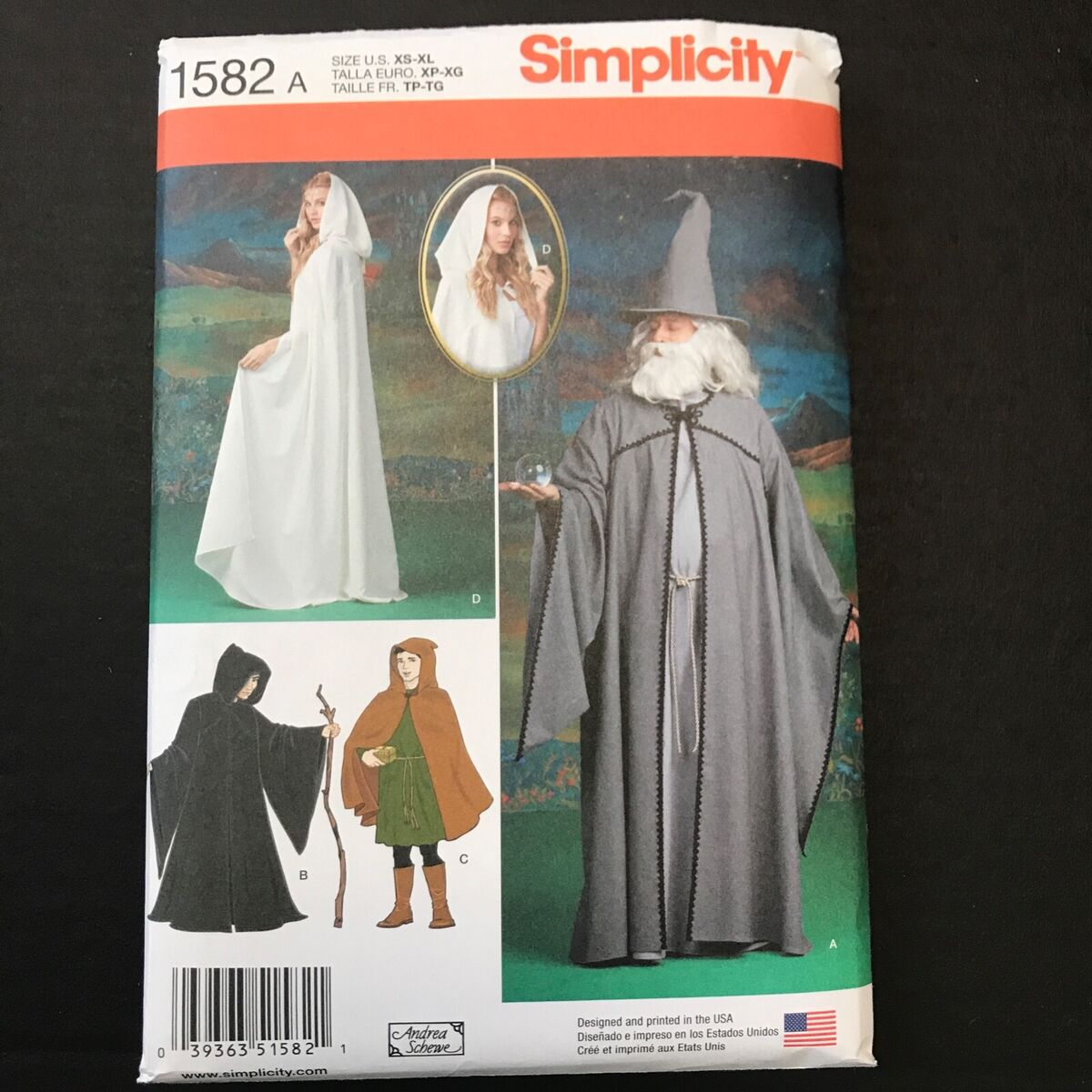The image depicts a sewing pattern packet set against a black background. The packet, labeled with the number 1582A and offering sizes from XS to XL, is from the brand Simplicity, which is prominently displayed in red text on the top right corner. Below the red text, a red stripe runs across the envelope, under which there are several photographs of models showcasing the different fantasy-style capes and costumes that can be created using the pattern. These capes include styles inspired by wizards, Little Red Riding Hood, and witches, with one model wearing a gray cape trimmed with black, complete with a matching wizard’s hat and white beard. Another model is dressed in a white, hooded maiden’s dress. The bottom left of the packet features illustrations of additional cape designs, such as a child in a brown cape with a green tabard, black leggings, and boots. The bottom section of the packet includes a black barcode, a watermark reading "Andrea Shewey," and a flag with the text "Designed and Printed in the USA."